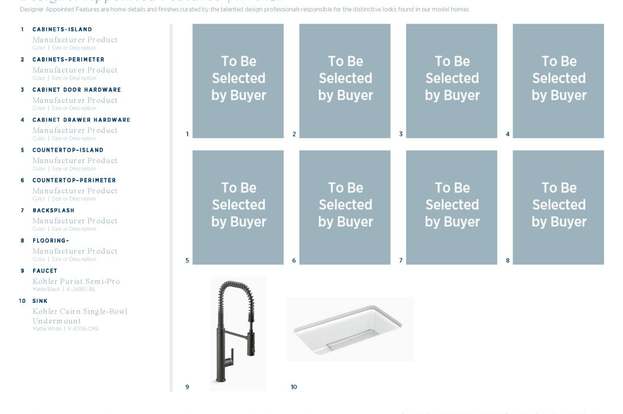The image depicts a website interface without any visible company name or URL. The background is predominantly white, with text transitioning from dark blue to light blue. On the upper left side, there are ten numbered rows:

1. **Cabinets Island** - Followed by descriptive text.
2. **Cabinets Perimeter** - Followed by descriptive text.
3. **Cabinets Dode Hardware** - Followed by descriptive text.
4. **Cabinet Drawer Hardware** - Followed by descriptive text.
5. **Countertop Island** - Followed by descriptive text.
6. **Countertop Perimeter** - Followed by descriptive text.
7. **Backsplash** - Followed by descriptive text.
8. **Flooring** - Followed by descriptive text.
9. **Faucet** - Followed by descriptive text.
10. **Sink** - Followed by descriptive text.

Dominating the center to right portion of the image are two rows, each containing four numbered squares (1-4 on the top row and 5-8 on the bottom row). Each square is labeled with the text "To be selected by buyer."

This detailed layout suggests an organized catalog for a selection process, likely related to home improvement or interior design.